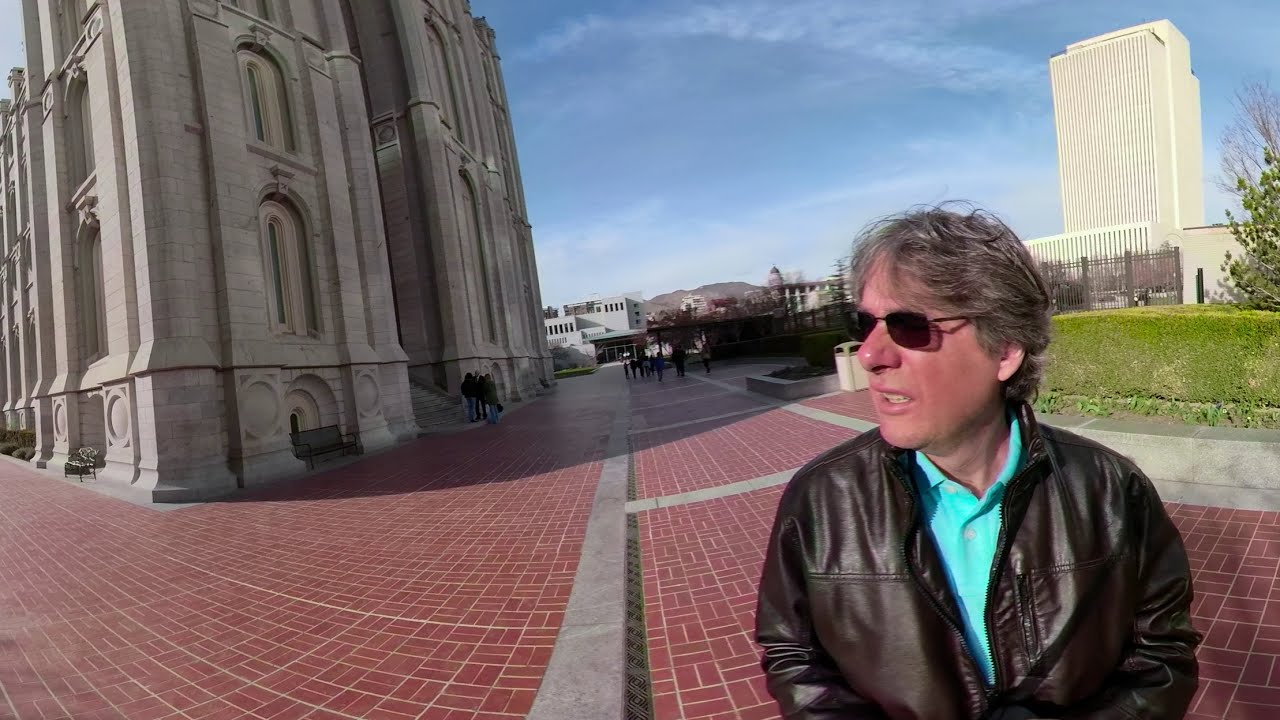The image depicts a man standing outdoors on a red brick ground interspersed with cement pathways. He is positioned in the right segment of the picture, wearing dark sunglasses, a turquoise polo shirt, and a black leather jacket. His grey hair appears tousled, and his face has a noticeable sunburn. He looks somewhat confused. Behind him, there's a large, foreboding gothic-style building made of grey cement, at least four stories tall, though the top is cut off in the picture. The setting seems to be a sunny day, evident from the bright blue sky and vibrant green grass and shrubbery surrounding the area. In the background, there are other buildings that resemble government structures, along with mountains visible in the distant background. The scene also includes several people who look like tourists, benches, a trash can, and a gated fence, giving it a touristy vibe.